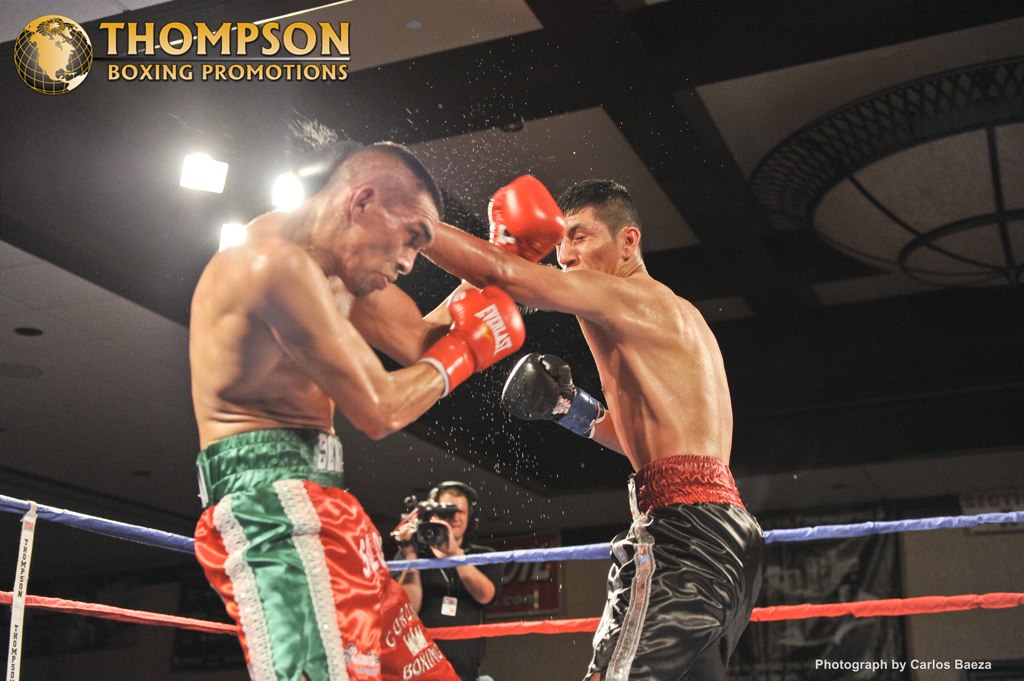The image captures an intense moment in a boxing match set in an indoor arena. The scene is framed by the top rows of blue and red ropes of the boxing ring, with a white and black tiled ceiling adorned with spotlights and a dome lamp above. Two boxers are fully engaged in the fight: the one in the foreground, a shirtless Caucasian with a shaved head, red gloves, and red, green, and white shorts, is taking a punch from his opponent. His opponent, possibly of Mexican descent, sporting short, dark wiry hair, black gloves, and black boxing shorts with a white stripe and red waistband, is delivering the punch with his left hand. The force of the punch is evident from the spray of sweat around the face of the boxer on the left. Both athletes are central to the composition, with a cameraman in a black shirt positioned in the background, capturing the action. The overall atmosphere seems dimly lit yet focused, with the details and dynamics of the match taking center stage.